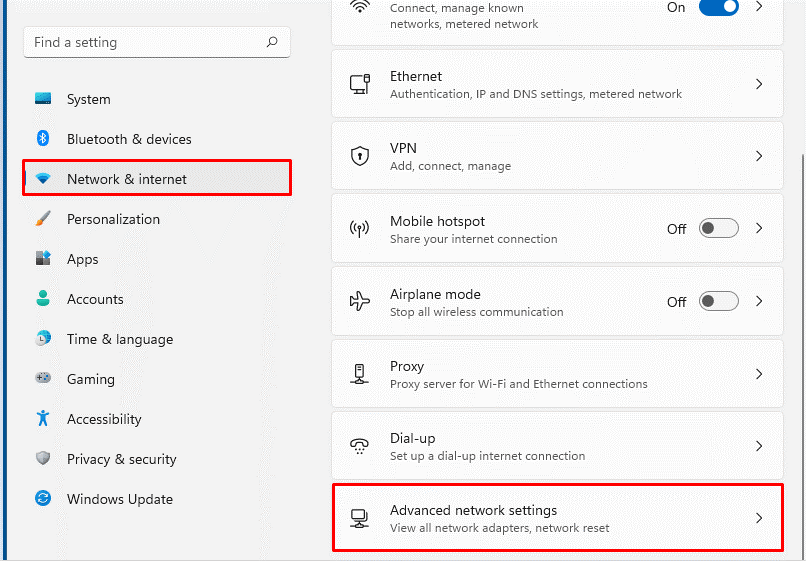This image depicts the settings interface of what appears to be either a tablet or a laptop, given the aspect ratio and layout. At the top-left corner, there's a 'Find settings' search bar encased in a rectangular box with a magnifying glass icon at the end. Below the search bar, the main settings categories are listed as follows:

1. **System**
2. **Bluetooth & Devices**
3. **Network & Internet** (This section is highlighted with a red-edged rectangle)
4. **Personalization**
5. **Apps**
6. **Accounts**
7. **Time & Language**
8. **Gaming**
9. **Accessibility**
10. **Privacy & Security**
11. **Windows Update**

Each category has an associated icon on its left-hand side.

On the right-hand side of the interface, under the 'Network & Internet' section, the following details are displayed:

- **Wi-Fi:** Lists 'Connect,' 'Manage known networks,' and 'Metered network,' with the latter being toggled on and an arrow to the right.
- **Ethernet:** Shows options for 'Authentication,' 'IP & DNS,' and 'Setting metered network,' each with a right arrow.
- **VPN:** Options include 'Add,' 'Connect,' 'Manage mobile hotspots,' and 'Share your internet connection,' with the hotspot sharing toggled off.
- **Airplane Mode:** This is toggled off.
- **Proxy:** No further details are provided.
- **Dial-up:** No further details are provided.
- **Advanced Network Settings:** Features 'View all networks,' 'Adapters,' and 'Network reset,' with this section outlined in a rectangle box and marked with a right arrow.

This comprehensive and well-organized interface outlines all essential settings and their statuses, aiding users in managing and customizing their device’s configuration.